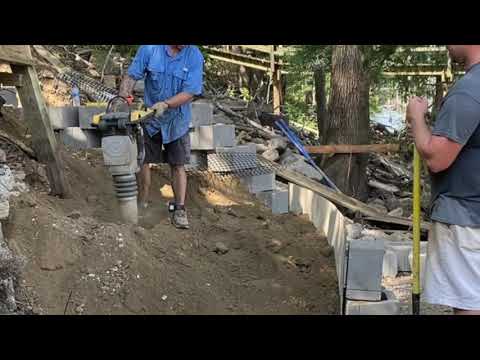The image depicts a construction site on an outdoor, dirt-covered incline that slopes upward from right to left. The scene features two men engaged in work amidst a cluttered background with various items like wood pieces and blue tulle scattered around. In the center of the image, a man in a blue short-sleeve button-down shirt, brown shorts, and tennis shoes is operating a gray tool that drills into the ground or a concrete post. This man's face is not visible because it is cut off by a black border at the top of the picture. To the far right, another man stands near a curved, waist-high wall of cinder blocks. He wears a dark gray short-sleeve shirt and white shorts, and is holding a yellow shovel or similar hand tool, with a hint of facial hair visible on the left side of his face. The background includes steps, a tree trunk, and what appears to be a bridge, suggesting an outdoor setting on what seems to be a warm, sunny day.